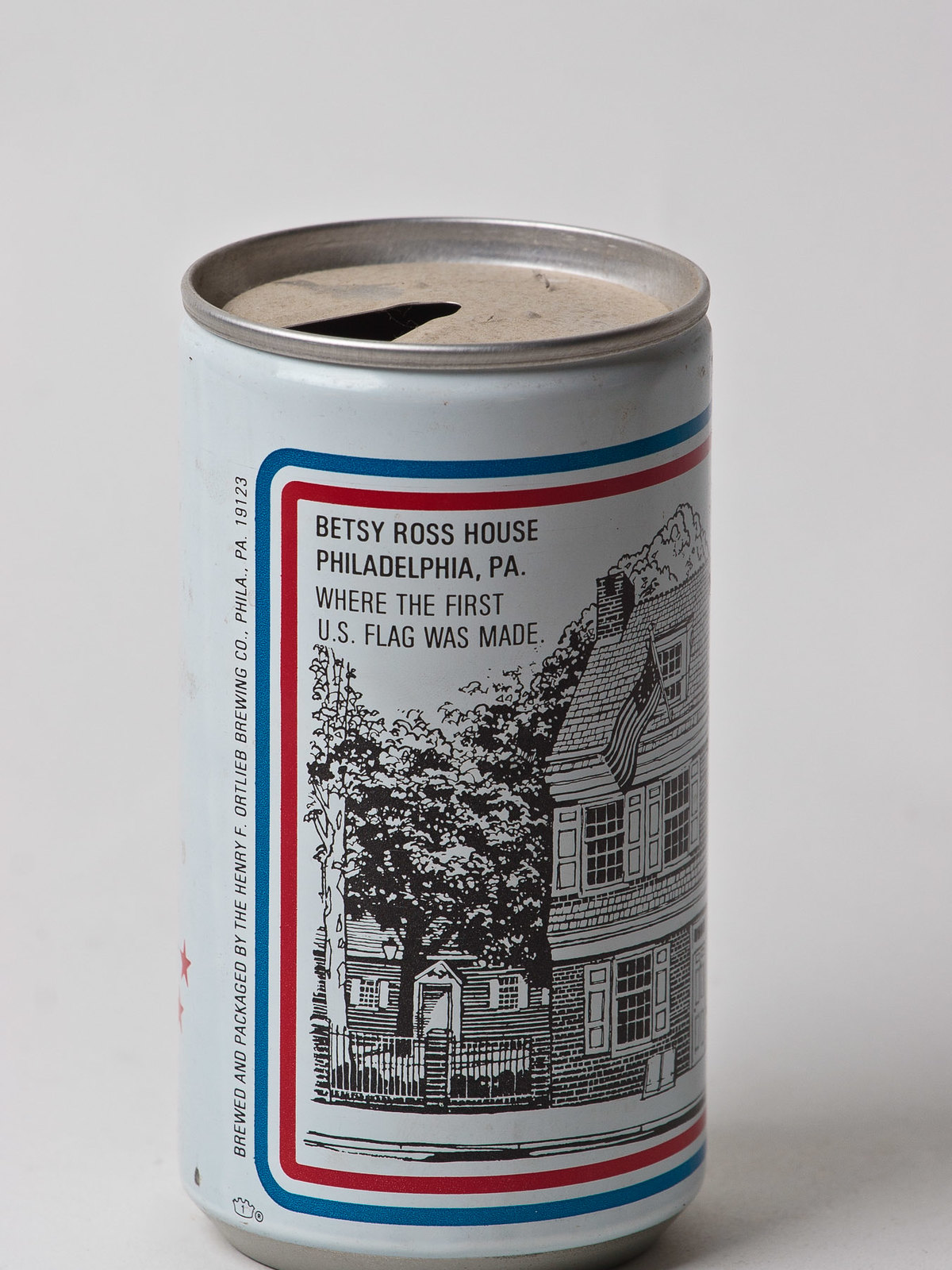The image depicts a white tin can with a distinctive design on its front. The central feature of the can’s design is a rectangle bordered by three lines—a blue line on the outer edge, a white line next, and a red line on the inside. The can commemorates the Betsy Ross House in Philadelphia, the historic site where the first U.S. flag was made. On one side of the can, there is a detailed line drawing of the Betsy Ross House, a tree, and another nearby house. Additionally, a small label indicates that the beer was brewed and packaged by the Henry F. Ortlieb Brewing Company in Philadelphia, complete with the zip code. The can shows signs of age and use, with the top appearing quite dusty and the can having been opened.